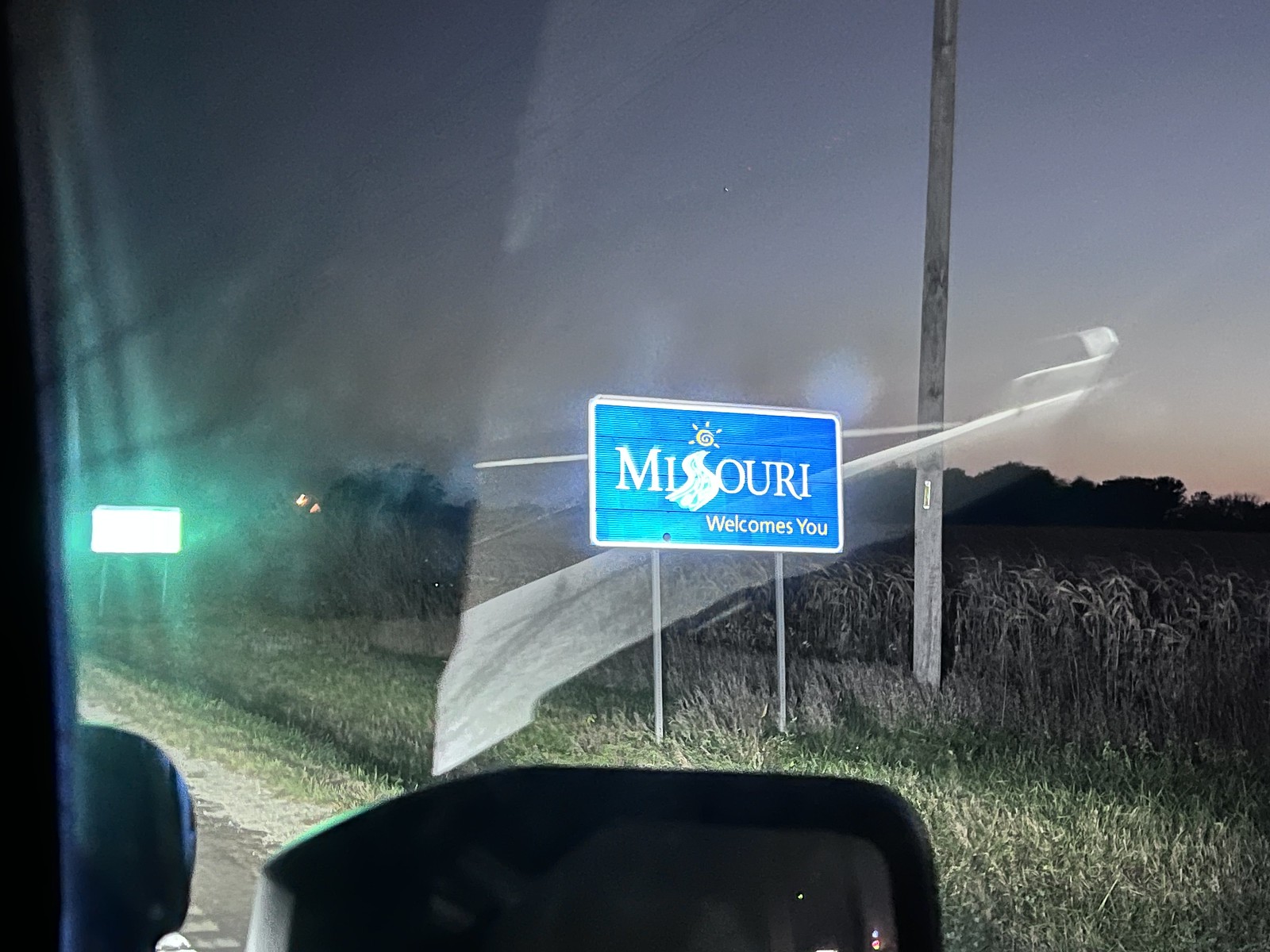This colored photograph, likely taken at early dawn or late sunset, captures a scenic moment through the windshield of a bus or RV. The primary focus is a rectangular road sign with a blue background, held up by two silver poles, showcasing white lettering that reads "Missouri" with a small sun graphic above the 'S'. Below the state name, the sign warmly states "welcomes you." To the right of the sign, a utility pole extends vertically out of the frame, set against a foreground of grassy terrain that transitions into a background of wilted corn stalks. The sky transitions from dark blue at the top to an orange hue towards the horizon, suggesting either sunrise or sunset. On the left side of the image, partially illuminated by the vehicle's headlights, a street sign is visible but unreadable due to the glare. At the bottom of the photograph, the large rectangular side mirror of the vehicle is partially cut off, while the window frame is discernible on the far left, contributing to the immersive perspective from inside the vehicle.